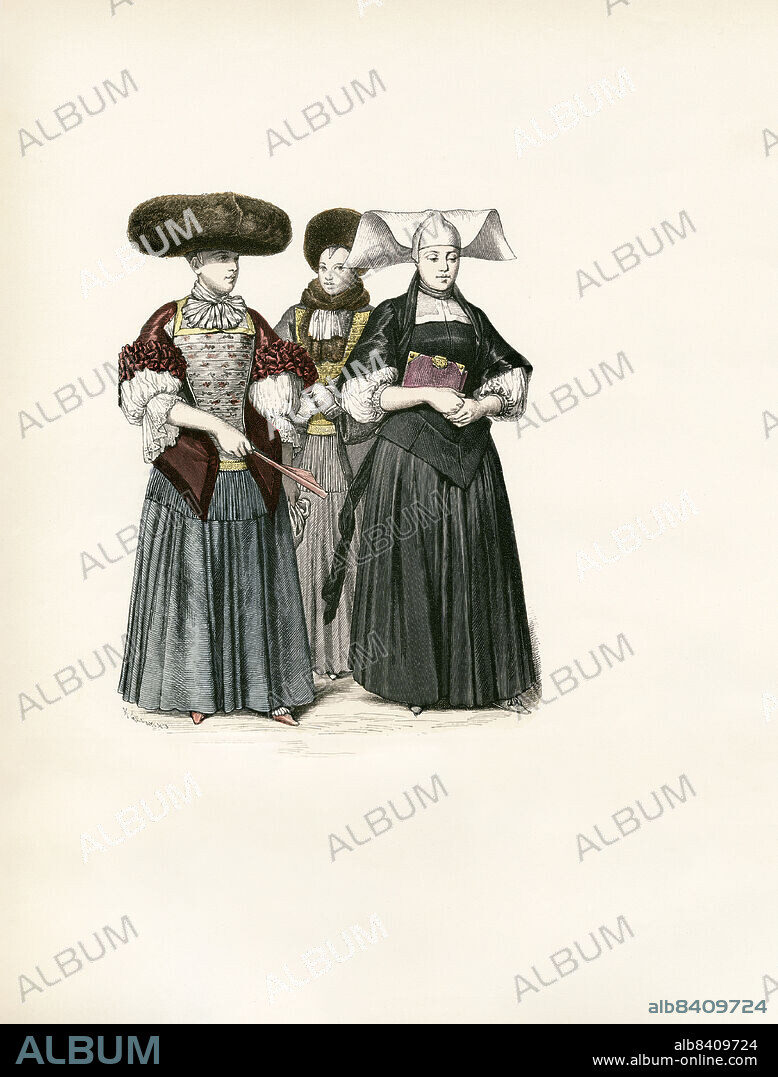The image features a detailed old-world style drawing of three women, reminiscent of 17th-century attire. Each woman stands out with distinct clothing and accessories against a gray background, overlaid with the word "album" repeated multiple times and accompanied by a watermark with the text "albumonline.com" and the code "ALB409724."

On the right, there's a woman in a dark green dress, holding a burgundy book with golden trim. She wears a white cap with flappy wings in the back, resembling a nun's habit. The woman in the middle is slightly obscured but identifiable by her gray dress paired with a golden vest and a brown scarf. She dons a round, bushy brown hat. The woman on the left is in a blue dress with a gray top and a burgundy vest draped over her shoulders and sleeves. She holds a red wand and wears a similarly large, round brown hat. Each woman's skin is fair, and their intricate attire is evocative of historical European fashion.